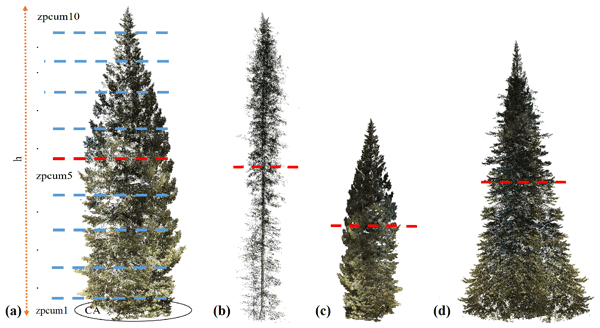The image features four distinct conifer trees, each labeled A, B, C, and D, set against a white background. On the left side, there's a vertical scale marked by an orange dotted line with double arrows pointing up and down, labeled ZPCUM10 at the top, ZPCUM5 in the middle, and ZPCUM1 at the bottom. Tree A, a green pine tree, is overlaid with a series of horizontal dashed blue lines, as well as a red dotted line intersecting it. Tree B, a skinny pine tree, has a single red-dotted line segmented into four parts and is labeled B at the bottom. Tree C has a similar red-dotted line segmented into five parts and is labeled C. The final tree, labeled D, also features a red-dotted line segmented into five parts.